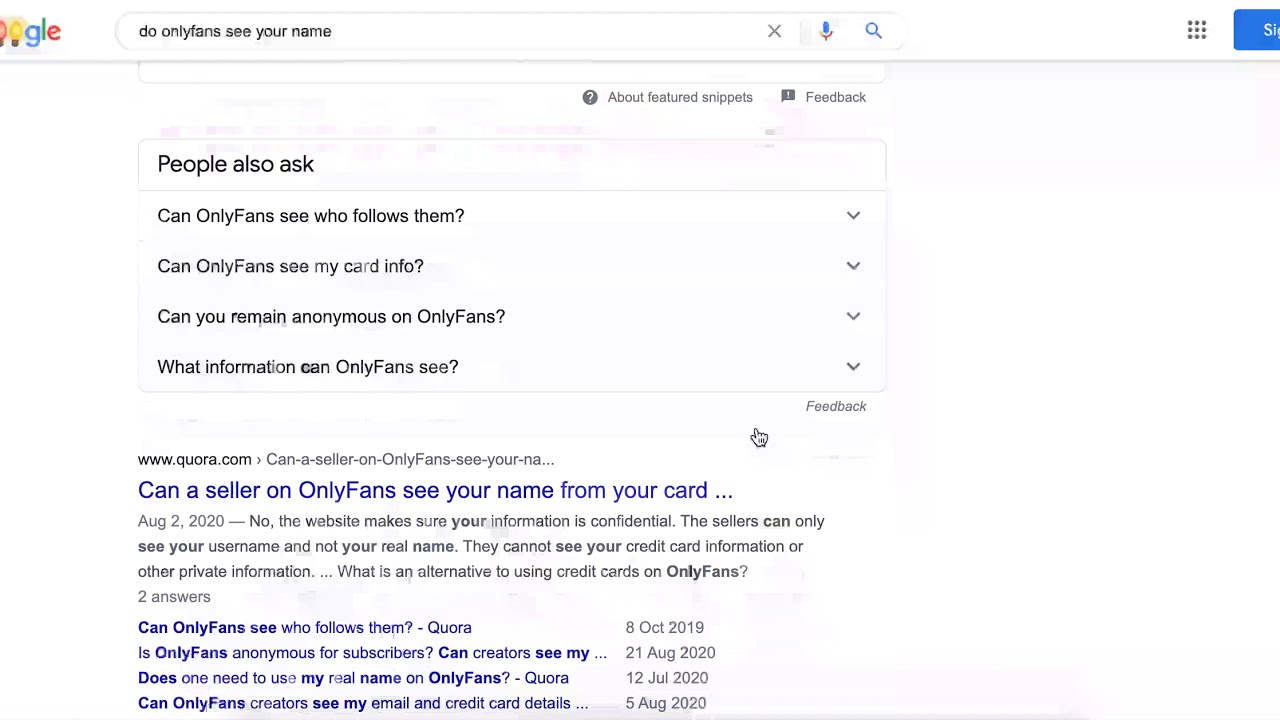This is a screenshot of a Google search results page. At the top left corner, the distinctive Google logo is clearly visible next to the prominent search bar. The search query entered into the bar reads: "Do OnlyFans See Your Name?" Below the search bar, there is a section titled "People also ask," displaying four related questions that users frequently inquire about concerning this topic. Beneath this section, the first web result appears, which is a link from Quora.com. If clicked, this link would lead to answers provided by Quora users addressing the question, "Do OnlyFans See Your Name?"